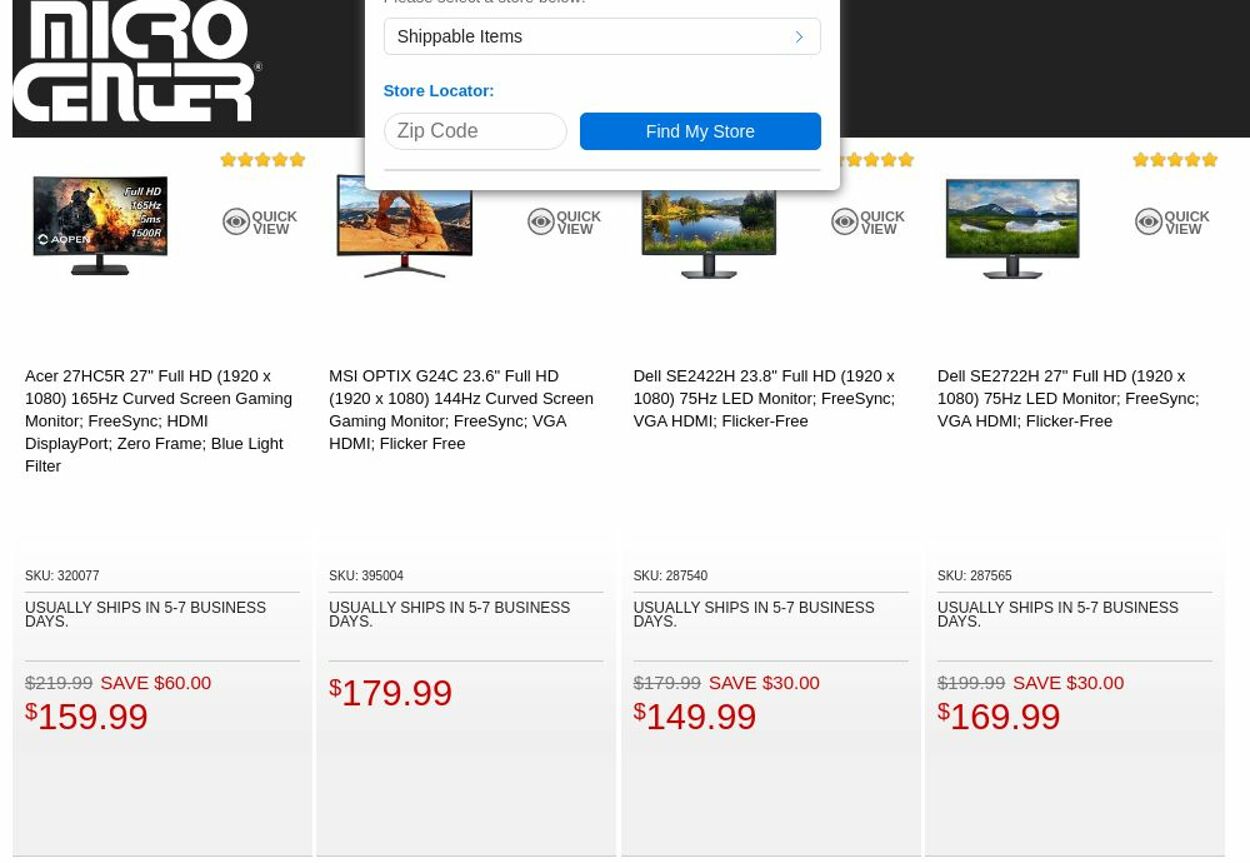The webpage displayed belongs to Micro Center and prominently features a user-friendly navigation bar at the top. This includes a dropdown menu labeled "Shippable Items" with an arrow indicating it can be clicked for more options. Additionally, there's a "Store Locator" section where users can input their zip code and click the "Find My Store" button to locate the nearest Micro Center.

Below the navigation bar, the page showcases a selection of computer monitors available for purchase. The first product is an Acer curved screen gaming monitor, equipped with FreeSync, HDMI display, zero frame, and a blue light filter. This monitor is currently discounted by $60, bringing its price down from $219.99 to $159.99.

The second option is an MSI monitor priced at $179.99. Following this, two Dell monitors are listed: the first is available for $149.99, down $30 from its original price of $179.99, and the second also offers a $30 discount, reducing the price from $199.99 to $169.99. The page notes that all these monitors can be shipped within five to seven business days.